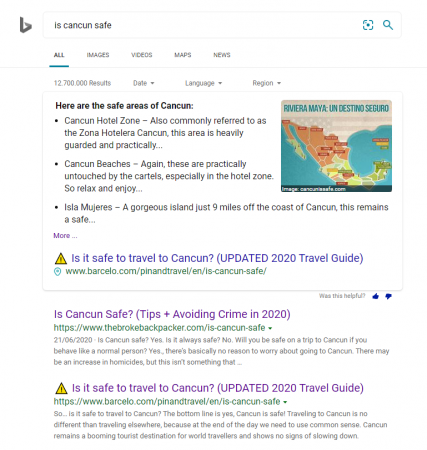Here is a cleaned-up and detailed caption for the image:

---

This image is a screenshot of a web search performed using an unidentified web browser. On the far left of the browser window, there is a three-dimensional, grey, triangular shape that is not fully complete. To the right of this shape, the search query entered is "Is Cancun safe?". Several tabs are visible below the search bar, labeled as "All", "Images", "Videos", "Maps", and "News", indicating this may be a Google search page. 

The search results are displayed prominently on the screen. At the top, a heading reads "Here are the safe areas of Cancun". Adjacent to this is a map titled "Riviera Maya, un destino seguro". 

Below this heading are bullet points detailing specific safe areas within Cancun:
1. **Cancun Hotel Zone (Zone Hotelera Cancun)**: This area is heavily guarded and particularly safe for visitors. The description trails off with an ellipsis.
2. **Cancun Beaches**: These beaches, especially within the hotel zone, are largely untouched by cartel activity, encouraging visitors to relax and enjoy.
3. **Isla Mujeres**: A beautiful island located just nine miles off the coast of Cancun, noted for its safety.

A "More" option suggests additional information can be accessed. 

Toward the bottom of the screenshot, there is a blue hyperlink titled "Is it safe to travel to Cancun? Updated 2020 travel guide," suggesting further reading. Two links below this title are already color-coded in purple, showing they have been previously opened. These links are titled "Is Cancun safe?" and "Is it safe to travel to Cancun?".

---

This detailed caption provides a clear and comprehensive description of the image, ensuring it is understandable even without the visual context.